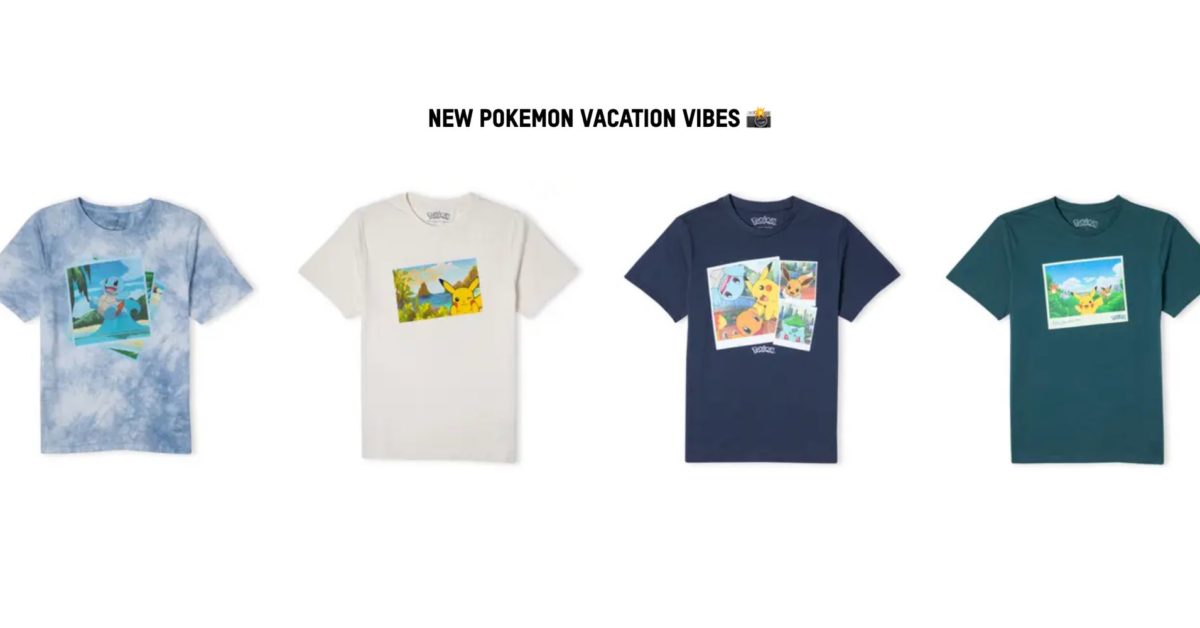This vibrant color image showcases a selection of four T-shirts arranged against a white background. All the T-shirts feature short sleeves and round necks, each adorned with distinct designs and white labels—except for the second T-shirt from the left, which sports a black label. Due to the image's framing, the far left and far right T-shirts are partially cut off, with only parts of their sleeves visible.

At the top of the image, black text reads "New Pokemon Vacation Vibes," accompanied by a small icon resembling a sunset with yellow hues over black.

Starting from the left:
1. The first T-shirt appears almost tie-dye in shades of grey and blue, featuring what may be a lake scene with a Pokemon character and surrounding greenery or potentially sky and trees—though the image detail is quite small.
2. The second T-shirt is white, adorned with a postcard design depicting a seaside scene. The scene includes a boat, some greenery, and a yellow Pokemon on the right, with perhaps another Pokemon in the middle of the postcard.
3. The third T-shirt is a very dark navy, showcasing two overlapping images of variously colored Pokemon. A larger Pokemon is on the left, while two smaller ones are on the right, accompanied by a white logo underneath.
4. The fourth T-shirt is dark green, featuring an image of a yellow Pokemon with a blue sky, clouds or mountains in the background, and greenery on either side.

Each T-shirt’s unique design captures the essence of "Pokemon Vacation Vibes," blending colorful graphics with serene, nature-inspired scenes.